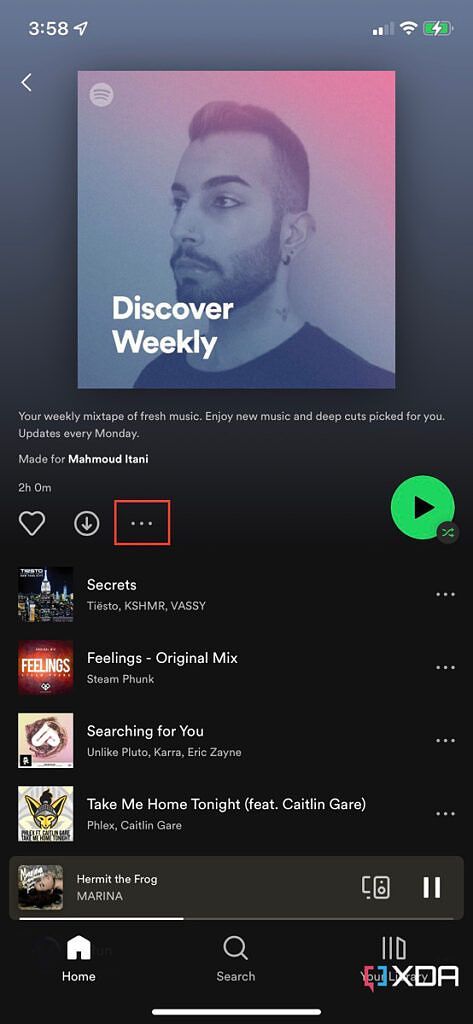Here is a cleaned-up and detailed caption based on the provided description:

---

**Screenshot of Mobile Device Displaying a Playlist on a Music Streaming App**

The image captures a screenshot of a mobile device featuring a playlist on a music streaming application. The current screen is primarily black, creating a sleek and modern interface. At the very top of the screen is a profile picture of a male, possibly a singer or performer, whose identity is not specified.

Above the profile picture, the header reads "Discover Weekly" in bold, inviting text. Directly beneath this, in smaller text, it elaborates, "Your weekly mixtape of fresh music, enjoy new music, and Deep Cuts picked for you. Updates every Monday."

Below this informative section, the interface displays a list of five recommended songs. For each song, there are three key elements displayed in a horizontal alignment: the song title, the name of the artist, and an illustration or album cover on the left. This visually appealing arrangement makes it easy for the user to browse through the new recommendations.

At the bottom of the screen, three navigation options are presented for user convenience: "Home," "Search," and "Your Library." These options allow the user to easily switch between different functions within the app.

The overall design is user-centric and visually organized, facilitating an efficient music discovery experience.